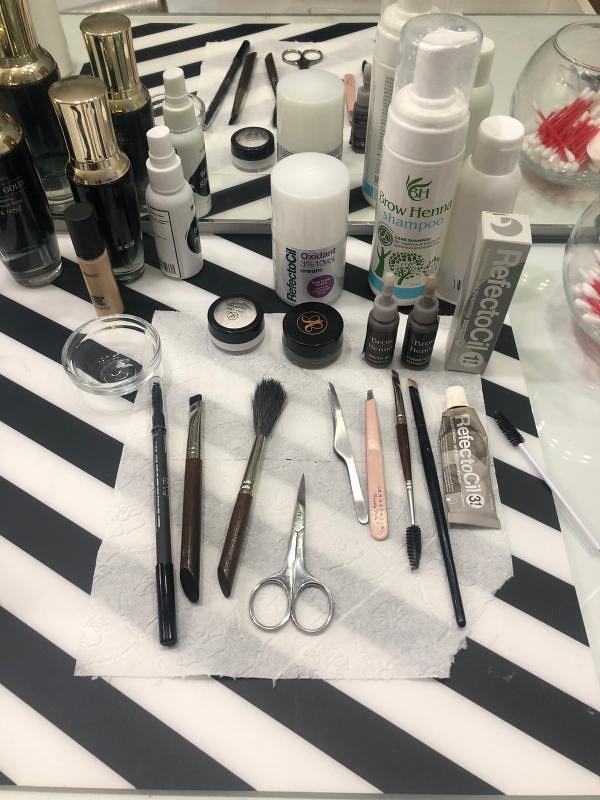This image showcases an assortment of skincare products and tools, meticulously arranged for a comprehensive display.

Starting from the top left, you can see sleek black cylinders adorned with silver caps. Positioned at the very back is a mirror that reflects the entire assembly in front of it, adding depth to the scene. Moving to the right, there’s a sophisticated silver cylinder along with some translucent latex gloves.

Next, there’s a brow henna shampoo bottle featuring a gray bottom section and a blue cylindrical top, capped with a clear cover and accompanied by a white cylinder nearby. On the extreme right sits a glass bowl filled with red-stemmed Q-tips, whose cotton ends are pristine white.

In the foreground, there is a white jar with a transparent cover accompanied by a black lid. Adjacent to this is a black container showcasing an intricate symbol. To its right lies a gray container followed by a ReflectoCil product, distinguished by its gray packaging with reflective lettering that emphasizes the brand.

Further right appears a thin stick equipped with a brush at its end, and nearby, a paintbrush with an elongated black handle. This brush sits next to an eyeliner brush.

On the far left side, there is a pink-handled tool with delicate metal tips, followed by tweezers. Nearby are a pair of scissors. Positioned next is a makeup brush with a black handle transitioning into a silver body, ending with a dense black bristle head. Finally, there’s a black pencil capped with silver, lying next to an undefined container.

Shadows cast by light create interesting patterns across the surface, enriching the visual complexity of the scene.